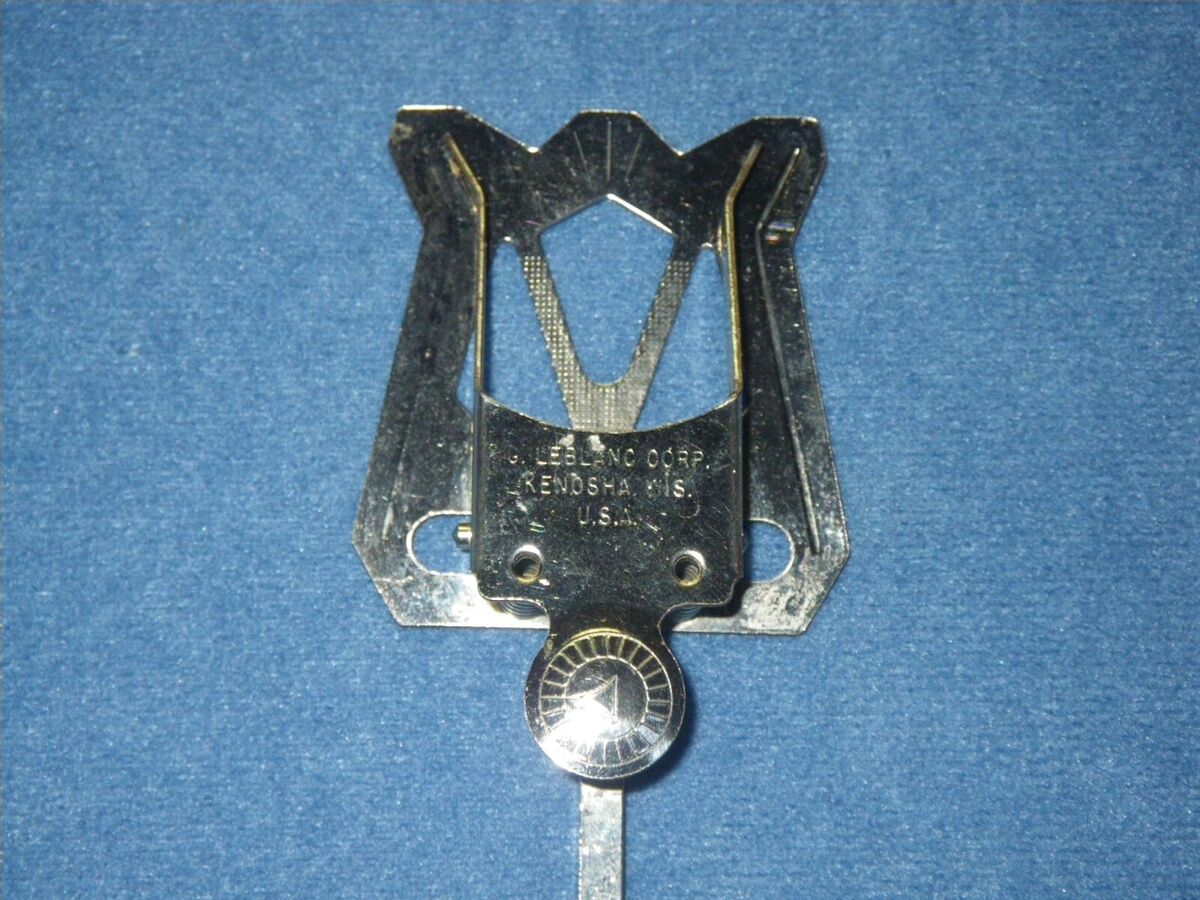The image depicts a metallic lyre attachment, designed for holding sheet music, set against a textured blue background that could be either cloth or a wall. The lyre, which is partially out of frame, shows a distinctive V shape at the top and transitions into prongs. At the front, it features an engraved inscription that reads "LeBlanc Corp., Kenosha, Wisconsin, USA," though the glow and glare in the photograph make the text difficult to discern. Below the inscription, there is a knob that can be tightened or loosened, presumably to secure the sheets of music. The metal object exhibits a shiny chrome finish with trapezoidal and ridge-like shapes contributing to its intricate design.